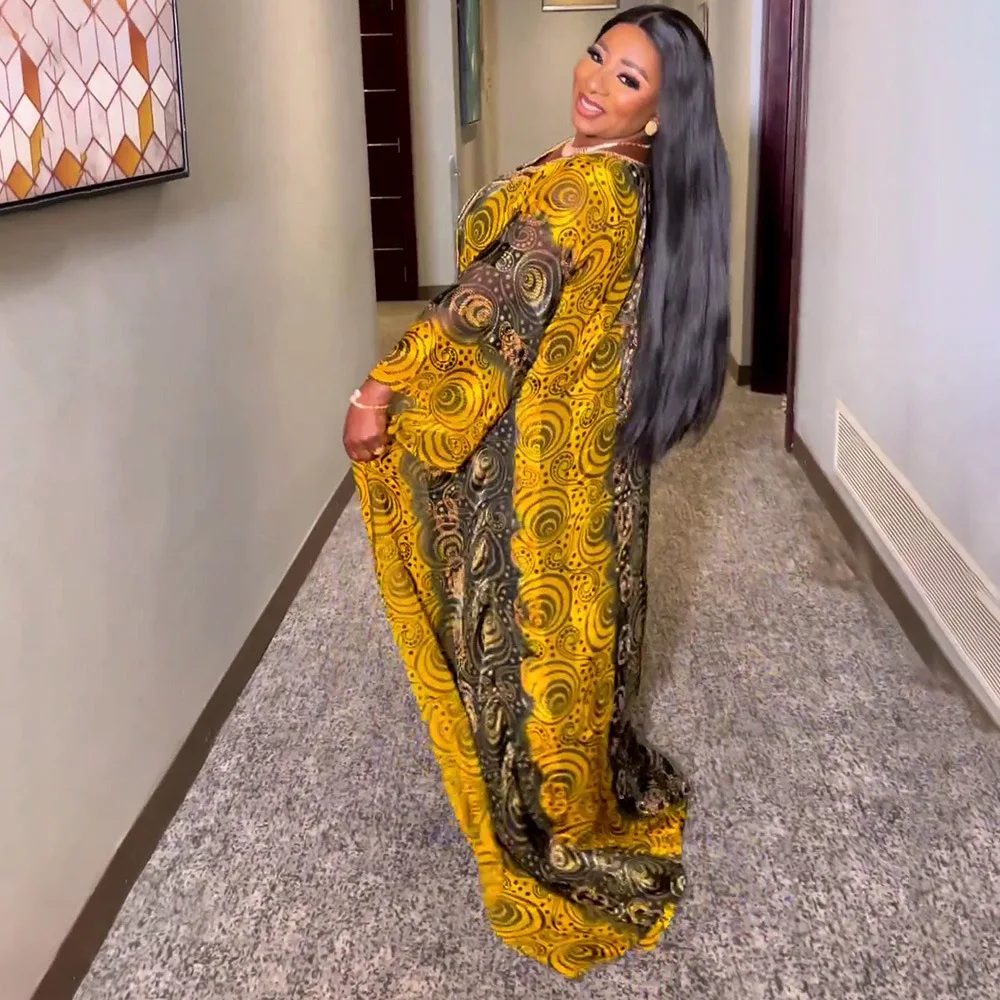This image features a striking African-American woman standing elegantly in a hallway. She exudes sophistication with her long, sleek black hair cascading to the top of her buttocks. Her dark skin is accentuated by subtle makeup, including red lipstick and black eyeliner. She is adorned with gold jewelry, including earrings, a bracelet, and possibly a gold or rose gold necklace.

The woman is wearing a floor-length, long-sleeved dress, which drapes gracefully around her. The dress is predominantly gold with wide black stripes, featuring intricate gold and black swirls, dots, and circles that imbue it with an ethnic flair. The swirls and patterns are uniformly distributed across the dress, creating a harmonious design.

She is positioned in the middle of a hallway with grayish walls and brown carpeting. In the background, a closed door is visible, with another door to the right and a secondary hallway to the left. There is also a vent on the wall and a partial view of a painting to the left.

The woman is turned slightly to her left, gazing directly at the camera with a serene and composed expression, showcasing her profile beautifully. This detailed portrait captures her elegant stance and exquisite attire, making her the undeniable focal point of the image.